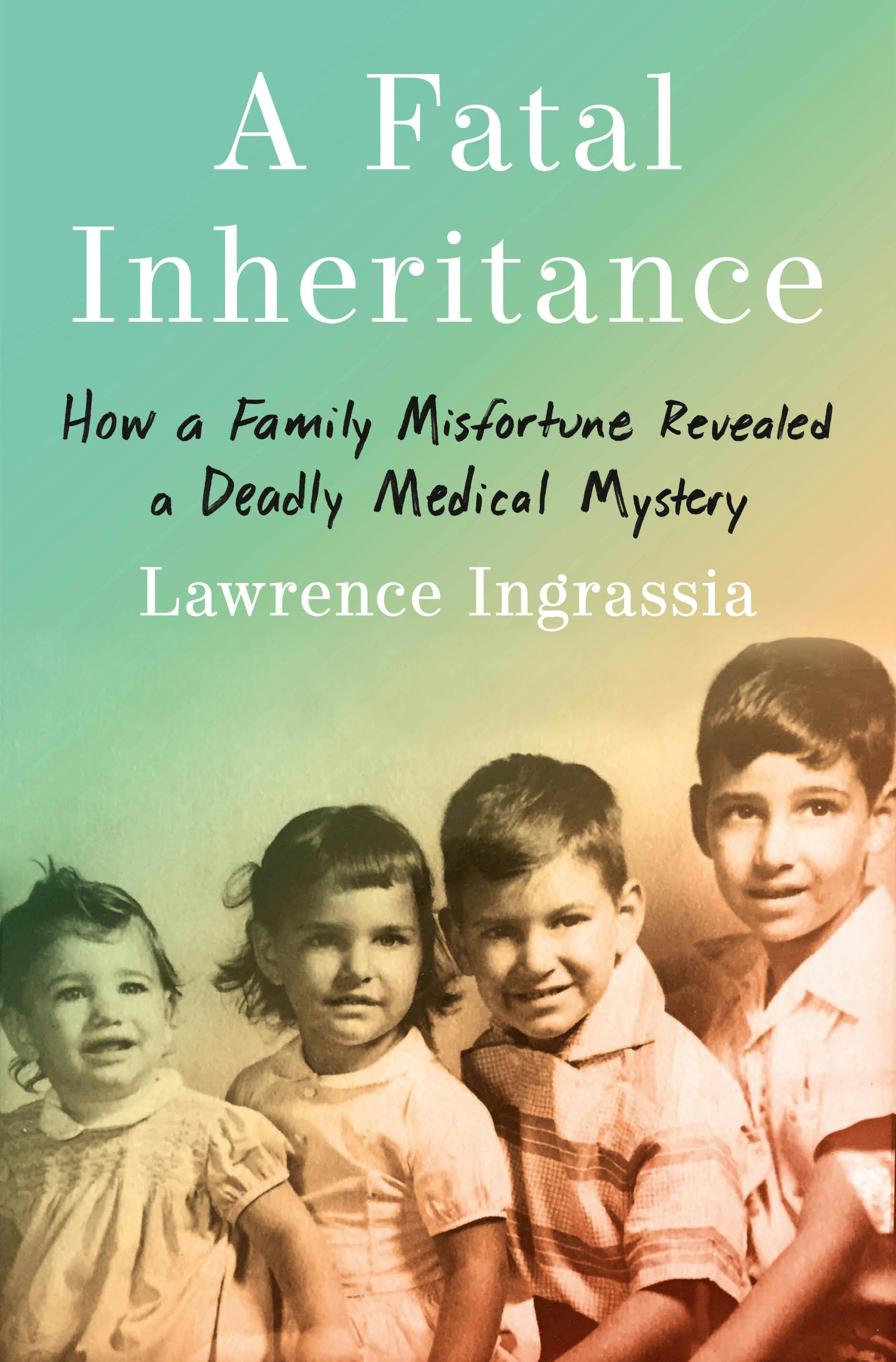The image depicts the cover of a book oriented vertically. The top of the cover features a light blue-green background that transitions to a lighter brown shade. The title, *A Fatal Inheritance*, is written in white, mixed-case letters. Below it, in black mixed-case letters, is the subtitle: *How a Family Misfortune Revealed a Deadly Medical Mystery*. The author's name, Lawrence Ingrassia, is also printed in white text. Beneath this text is a black-and-white photograph of four children arranged in a stair-step fashion from left to right, with the youngest on the left and the oldest on the right. The two girls are positioned on the left, with the younger girl appearing to cry and wearing a blouse dress with short, straight hair. The older girl, next to her, has bangs and short hair tucked behind her ears, dressed in a whitish dress with buttons and a collar. To their right are two boys. The younger boy, smiling slightly, is wearing a collared striped shirt. The oldest boy stands behind him, with a similar hairstyle and a collared shirt, mouth slightly open. The children seem to be posing for a formal family photograph.